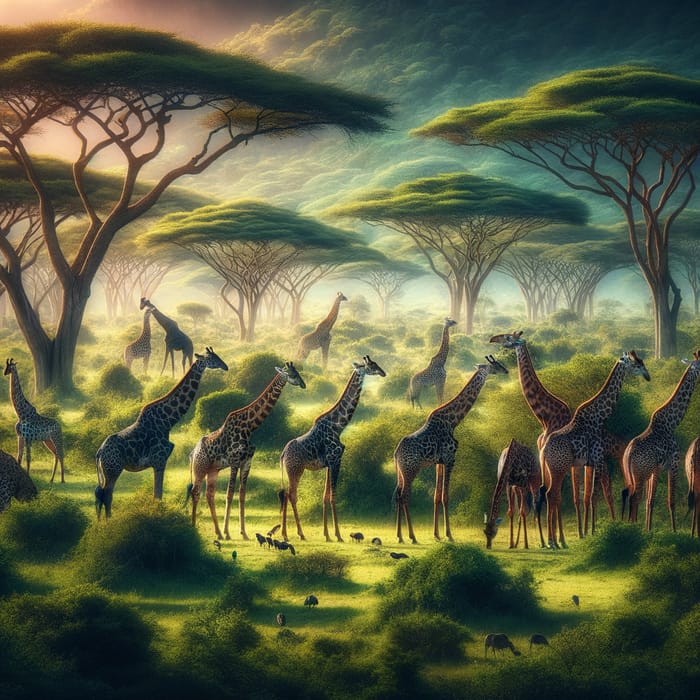The detailed computer-generated image, which resembles a colored pencil artwork, portrays an African safari scene rich with natural elements and animal life. At the forefront and center of the image, a large herd of giraffes—approximately 12 to 15—are gathered, their long necks falling short of the foliage of the acacia-like trees above them. Some giraffes are depicted with their necks bent down, seemingly grazing. Accompanying the giraffes are various smaller, indistinct animals and birds, with a few birds seen foraging on the ground and others perched in the trees. The landscape features green grass and dispersed circular green bushes, giving a lush appearance to the savanna setting. The trees, known for their umbrella-like shape with branches that stretch high and spread out at the top, are indicative of the African environment. The background reveals a large, partially cropped mountain adorned with green bushes, shrouded in a haze or fog, enhancing the depth of the scene. A ray of light penetrates from the top left, illuminating parts of the ground. The overall style of the image leans towards photorealism, capturing fine details such as the light effects and the diverse fauna.